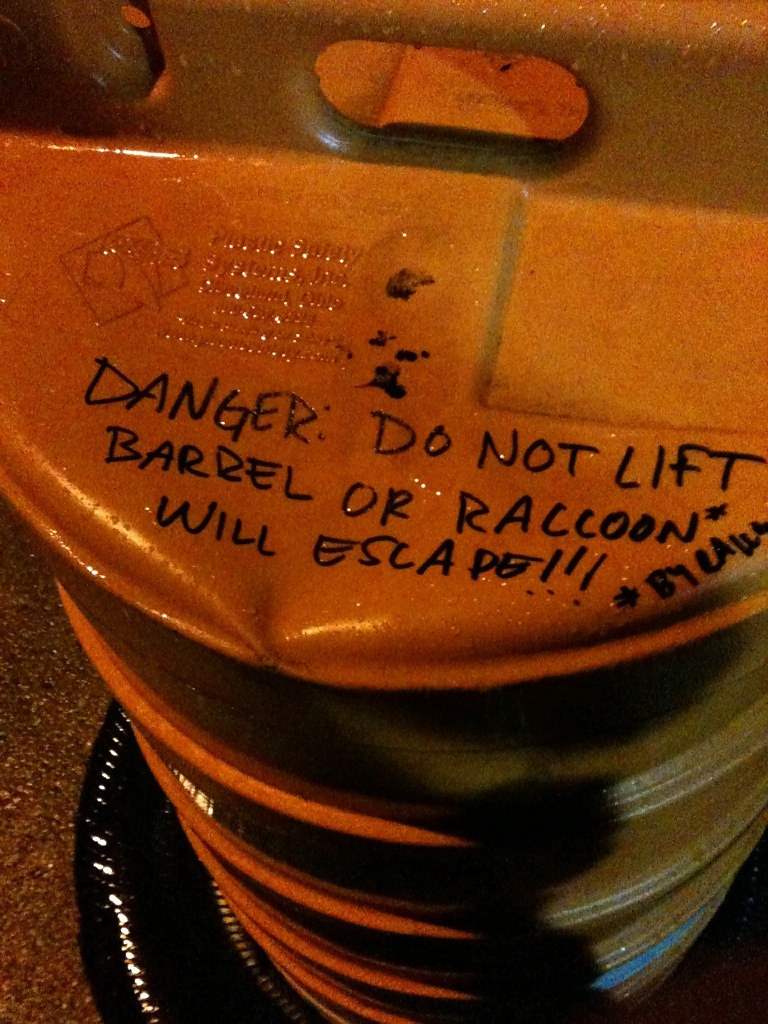The image presents a detailed close-up view of a cylindrical metal drum taken from above. The drum is predominantly orange with traces of yellow, suggesting it may have an orangish-red hue. A notable feature on the drum’s top is a handwritten message in black Sharpie marker that reads: "Danger, do not lift, barrel or raccoon will escape!!!" The handwriting appears casual and informal. The drum also has a shiny, black base, which likely aids in its stability. The surrounding ground, which appears brown and wet, suggests recent rain, further accentuating the drum’s moist surface.